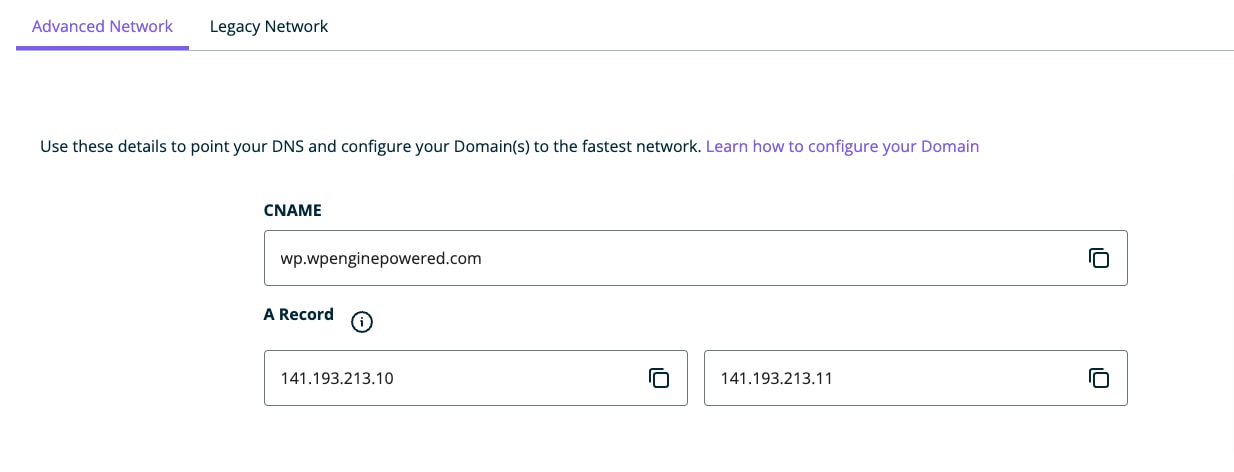Screenshot displaying a backend URL configuration section for a website:
- The entire interface has a clean, minimalistic design with a white background and black text.
- At the top of the screenshot, two options are visible: "Advanced Network" and "Legacy Network." The "Advanced Network" option is selected, highlighted in purple with a faint gray underline indicating the selection.
- Below this, a message in the text reads: "Use these details to point your DNS and configure your domains (or domain) to the fastest network."
- There is a clickable text in purple that states: "Learn how to configure your domain."
- The configuration details are divided into two sections:
  - The first section is labeled "CNAME" in bold. It features an input box filled with the text "WPenguinPower.com" and an adjacent icon with a 'copy' symbol for easy copying.
  - The second section is labeled "A record" in bold. It contains one input box displaying the IP address "141.193.213.10" and another input box with a different IP address.

This caption provides an in-depth description of the elements within the screenshot, highlighting the purpose and details of the DNS configuration options.